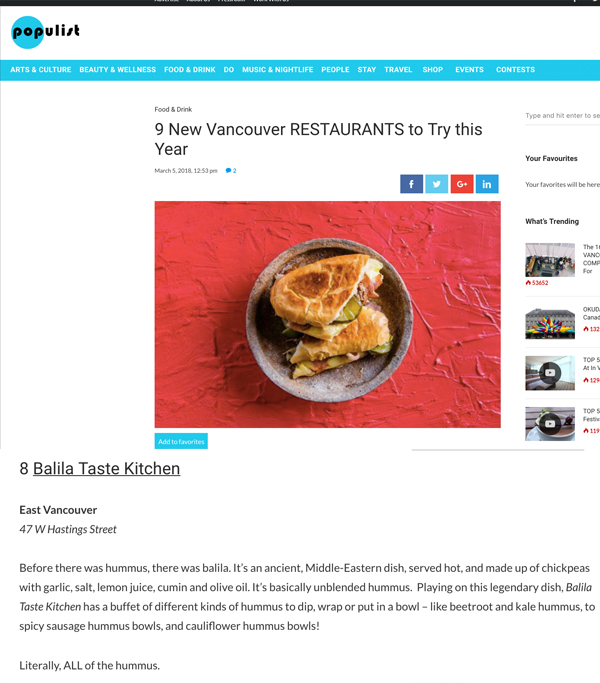Screenshot Description: 

The screenshot showcases content from the platform "Populist" with the name clearly spelled out in the background. The first three letters, "P-O-P," are placed within a blue circle. It focuses on "Food and Drink" and emphasizes "non-New Vancouver restaurants," with the word "RESTAURANTS" appearing in all capital letters.

At the center of the image, there is a visually appealing photograph of a sandwich resembling a panini. This sandwich rests on what seems to be a stone bowl. The backdrop of the image features a red surface, possibly a wall or floor, giving the whole scene a vibrant ambiance.

Above the photograph, there are icons for several social media platforms: an "F" for Facebook, a bird for Twitter, a "G" for Google, and "I-N" for LinkedIn.

Adding more context, the image includes the text: "Balila Taste Kitchen, East Vancouver, 47 West Hastings Street." It also mentions, "Before there was Hummus, there was Balila," giving a nod to the origins of a traditional dish known as Balila.